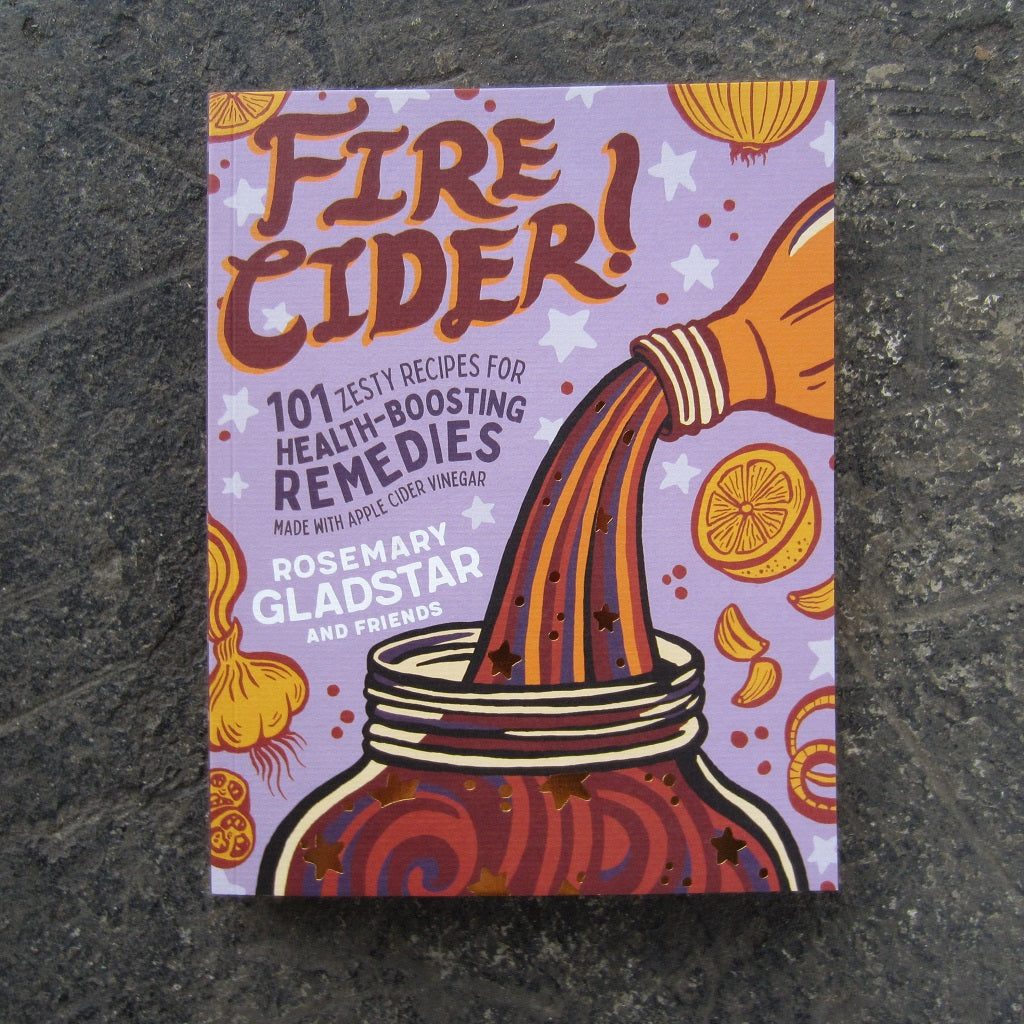The image depicts the cover of a small hardcover book titled "Fire Cider: 101 Zesty Recipes for Health-Boosting Remedies Made with Apple Cider Vinegar, Rosemary Gladstar, and Friends." The background of the cover is a rich purple, adorned with several white stars and stylized images of various food items, including lemons, garlic, onions, and onion rings, illustrated in yellowish and orange hues. Prominently featured on the cover is a detailed, cartoonish depiction of apple cider vinegar being poured from a bottle into a clear jar, shown in vibrant, repeated colors of red, purple, and orange, blending into a gooey mix. The text of the title is in dark red with an exclamation point, following a curvy design with blue for the main title and white for the authors' names. The book lies on a gray, stone-like background that may resemble a countertop or tiled surface, adding to the overall vivid and dynamic presentation.